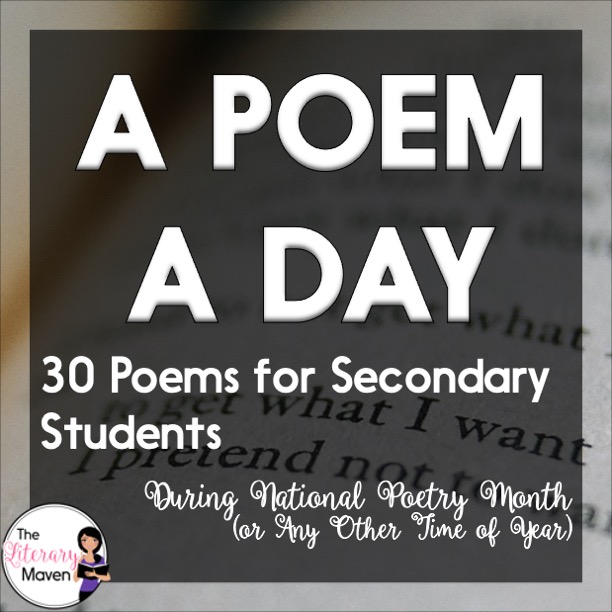The image is a graphic design with a light gray to tan gradient border. The central portion appears to be a photograph featuring a close-up of book text, though the text itself is not distinguishable. Dominating the image, in solid white, all-caps font, are the words "A POEM A DAY." Just below this, in smaller, mixed-case font, it reads "30 Poems for Secondary Students." Beneath that, written in elegant white cursive, is the phrase, "During National Poetry Month (or any other time of year)." In the bottom left corner, there is a circular logo. Inside the circle, there is a clipart-style image of a woman with long black hair wearing a purple shirt, holding a book in her left arm. Adjacent to the woman, the text reads "The Literary Maven" in a combination of black and pink cursive fonts. This graphic appears to be an advertisement, possibly aimed at promoting National Poetry Month, and could be used on various digital platforms like websites or social media.